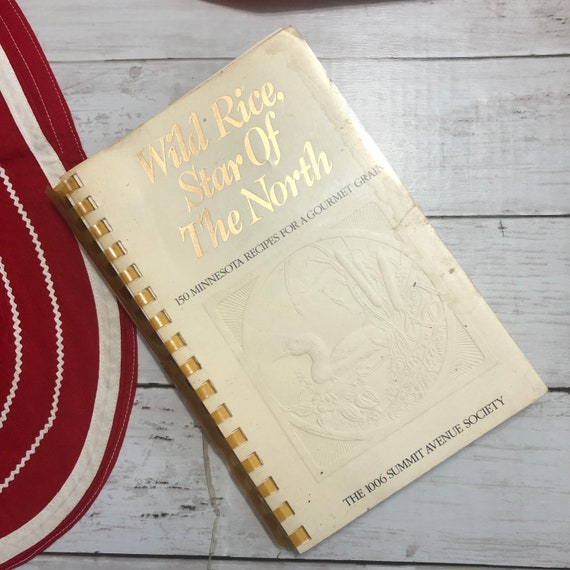The image depicts a rustic, whitewashed wooden table. At an angle on this table sits an off-white book with a yellow, plastic comb binding. The book's cover features large, italicized gold text reading: "Wild Rice, Star of the North." Beneath this, the subtitle in smaller black text states: "150 Minnesota Recipes for a Gourmet Grain." Toward the bottom, it reads in small black letters: "The 1006 Summit Avenue Society." The center of the cover showcases an embossed image of a duck in a pond, surrounded by cattails and wild plants. To the left of the book, an edge of an oval-shaped, red-and-white-striped placemat with white rickrack detail is visible. The setting of the book and placemat on the table creates a vintage, weathered look.